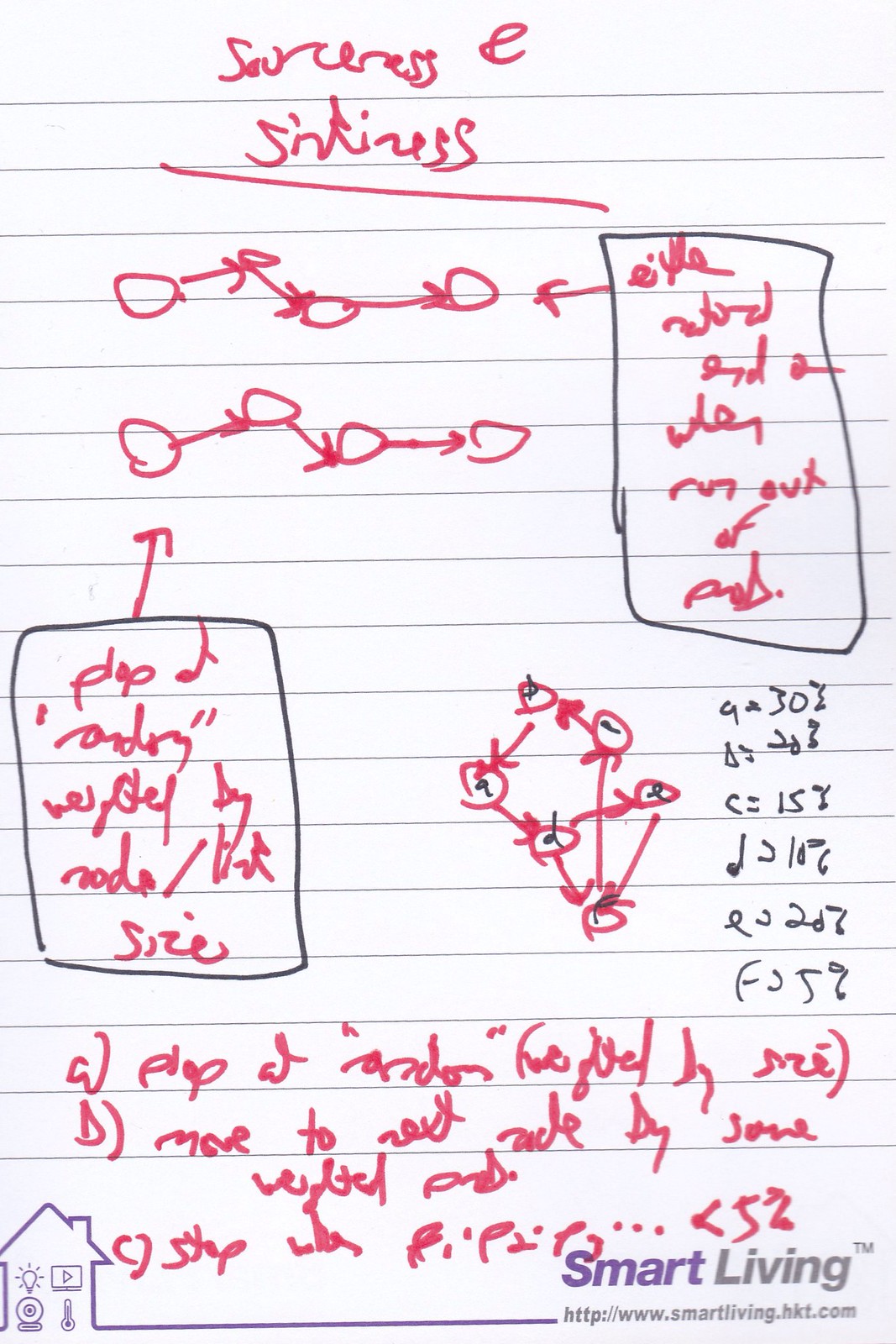This vertical image features a handwritten note on white-lined paper, taken from a Smart Living notepad. The page contains both text and illustrations, created using red and black ink. At the top of the page, a partly legible heading appears to reference themes of success and sickness. The content includes four circles connected by arrows, suggesting a form of process or relationship, juxtaposed with vertically aligned rectangles drawn in black ink. Additionally, there are various letters paired with numbers scattered throughout the note. The bottom section of the page lists items A, B, and C, each accompanied by further handwritten notes. The Smart Living notepad's logo, a house icon, is visible in the lower left corner, while the brand's name and website are located in the lower right corner.